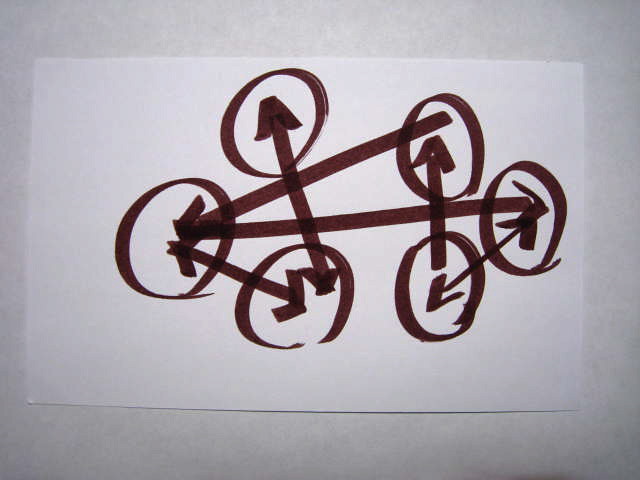In this image, a piece of white copy paper is placed against a grayish white backdrop, featuring an arrangement of dark maroon circles and lines drawn with a marker. There are six circles in total, with three on each side of the paper. These circles are interconnected by thick lines that mostly end in arrowheads. Particularly, the top circle on the right side connects to the middle circle on the left. The middle circle on the left also links to the middle circle on the right. Additionally, an arrow on the left side connects the top and bottom circles. The overall layout resembles a network or flowchart, where the arrows indicate the direction of connection between the circles.